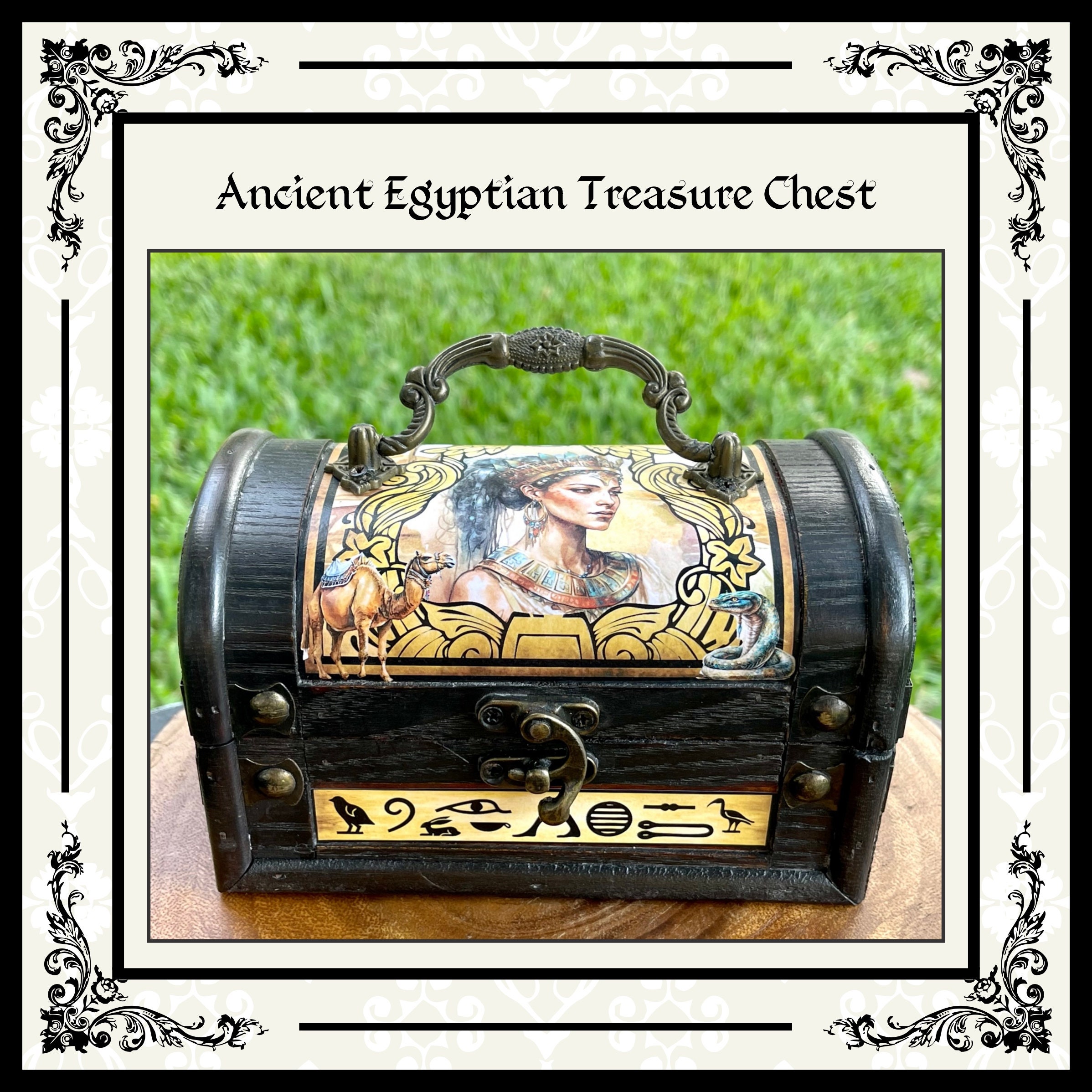The image is a detailed digital photograph depicting a small, black chest that resembles an old-style lunchbox. The chest, labeled "Ancient Egyptian Treasure Chest" in text positioned within a thick white border at the top, features ornate Egyptian designs with an illustration of a woman on the lid and additional symbols on a thin horizontal rectangle on the side. The chest also has an ornate handle and a lock on the front. It is placed on a brown wooden surface with grass visible in the background. The entire photograph is framed with multiple decorative borders, including a thin light border, an outer black border with 19th-century style plant-themed emblems in each corner, and an overall thicker black border surrounding the entire image. The color palette of the image includes blacks, greens, yellows, whites, blues, and golds.